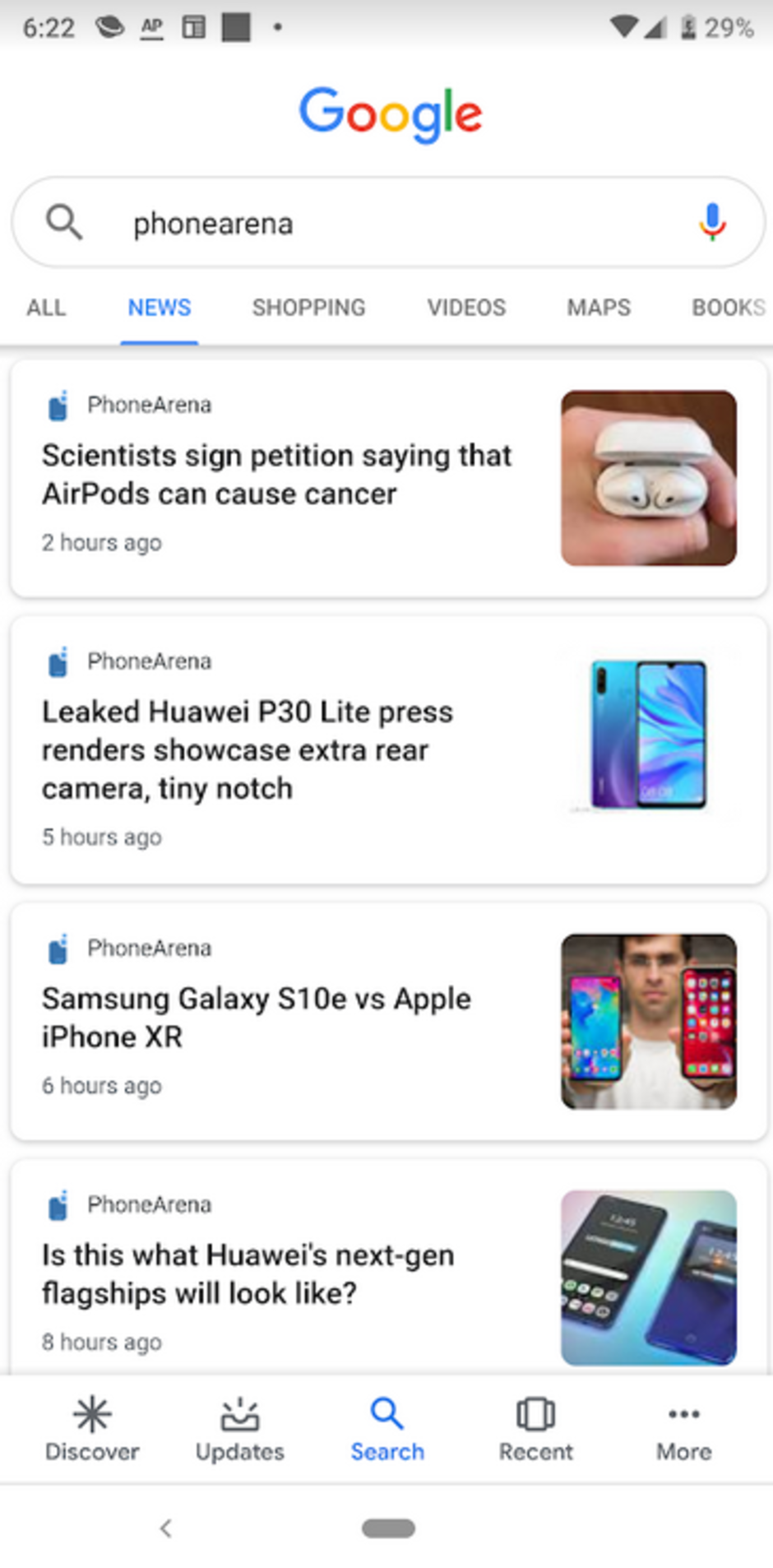The screenshot displays a mobile device interface. In the top-left corner, the device time is shown as 6:22. The status bar includes several icons: on the top right, you see a Wi-Fi connection symbol, a network signal bar, and a battery indicator showing 29% remaining. Below the status bar, there is a search box with "Phone Arena" typed in it. Above the search box, the Google logo is prominently displayed in its traditional colors: blue, red, yellow, blue, green, and red.

The screenshot also lists categories such as All, News, Shopping, Videos, Maps, and Books. Following these categories are several headlines from Phone Arena: 
1. "Scientist signed petition saying that airports can cause cancer" - posted two hours ago.
2. "Leaked Huawei P30 Lite price renders showcase extra rear camera, tiny notch" - posted five hours ago.
3. "Samsung Galaxy S10e vs Apple iPhone XR" - posted six hours ago.
4. "Is this what Huawei's next-gen flagships will look like?" - time of the post is not specified.

The interface appears to be a typical news feed or article listing within a mobile browser or application.